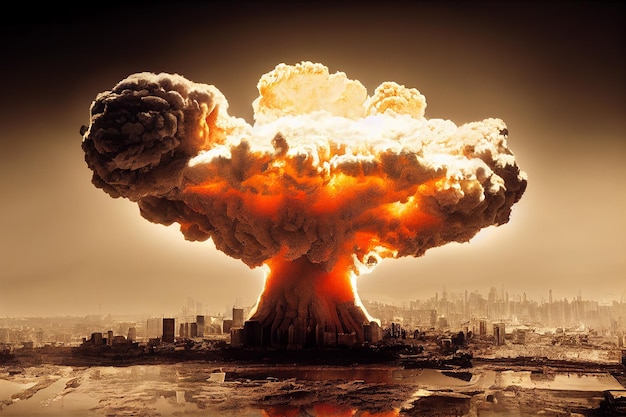This captivating digital creation depicts a horrifying atomic bomb explosion amidst a densely packed city skyline. The square image, devoid of borders and set against a predominantly dark background, captures the stark contrast between the vivid, multi-colored explosion and the otherwise dim surroundings. The upper corners of the image are cloaked in black, transitioning to brownish hues that frame the scene. Dominating the center, a colossal mushroom cloud—rendered in fiery oranges, reds, bright yellows, and an array of grays and blacks—rises ominously above the multistory buildings, making them appear minuscule in comparison. The explosion illuminates the dark sky, casting a surreal, almost otherworldly light over the area. At the very bottom, there appears to be a water harbor, adding a final touch of realism to this digitally crafted nightmare. The photograph, taken from a distance and elevated vantage point, highlights the scale of the devastation, making it a haunting and unforgettable image.